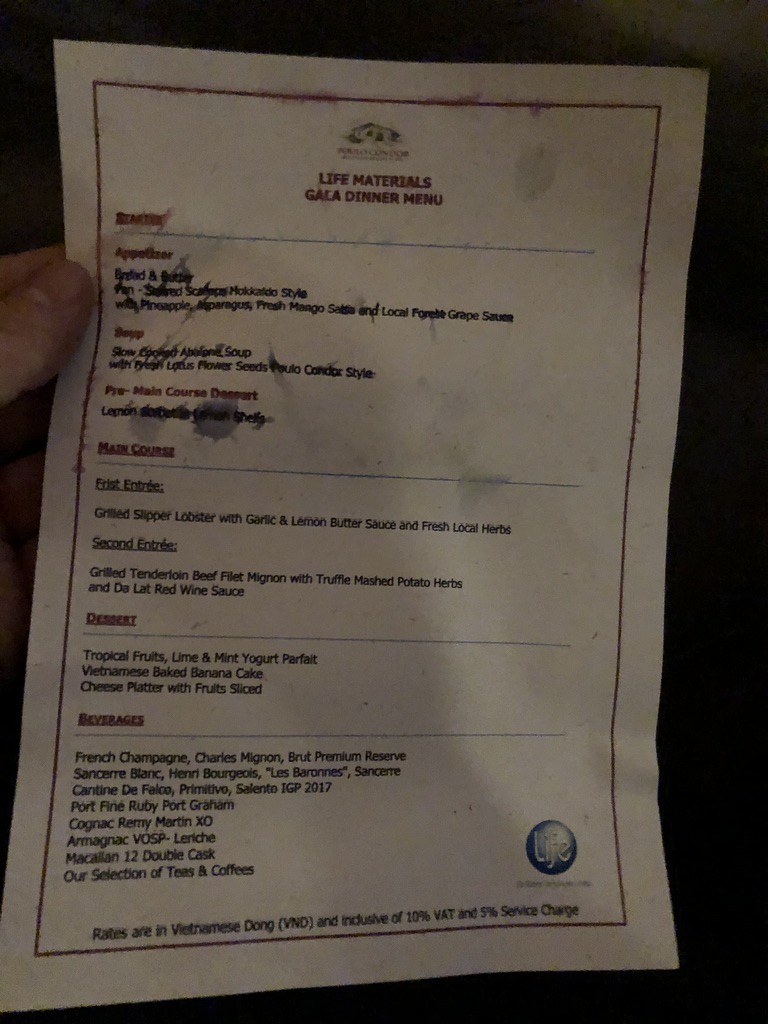In this grainy and slightly blurred photograph, a hand is seen holding a paper menu, which appears to have been wet and smeared. Despite the damage, the text on the menu is still partially legible. It reads:

**Chef's Materials Gala Dinner Menu**

**Appetizer:**

**Main Course:**

- **First Entree:** Grilled Slipper Lobster with Garlic and Lemon Butter Sauce, garnished with Fresh Local Herbs
- **Second Entree:** Grilled Tenderloin Beef Filet Mignon served with Truffle Mashed Potatoes and Herb-infused Dallotte Red Wine Sauce

**Dessert:**

- Tropical Fruits
- Lime and Mint Yogurt Parfait
- Vietnamese Baked Banana Cake
- Cheese Platter with Sliced Fruit

**Beverages:**

- French Champagne: Charles Mignon Brut Premium Reserve
- Sancerre Blanc: Henri Bourgeois, Les Barons Sancerre
- Port Fine Ruby: Port Graham
- Cognac: Remy Martin
- Armagnac: VOSP La Riche
- A selection of teas and coffees

**Note:** Rates are in Vietnamese Dong and inclusive of 10% VAT.